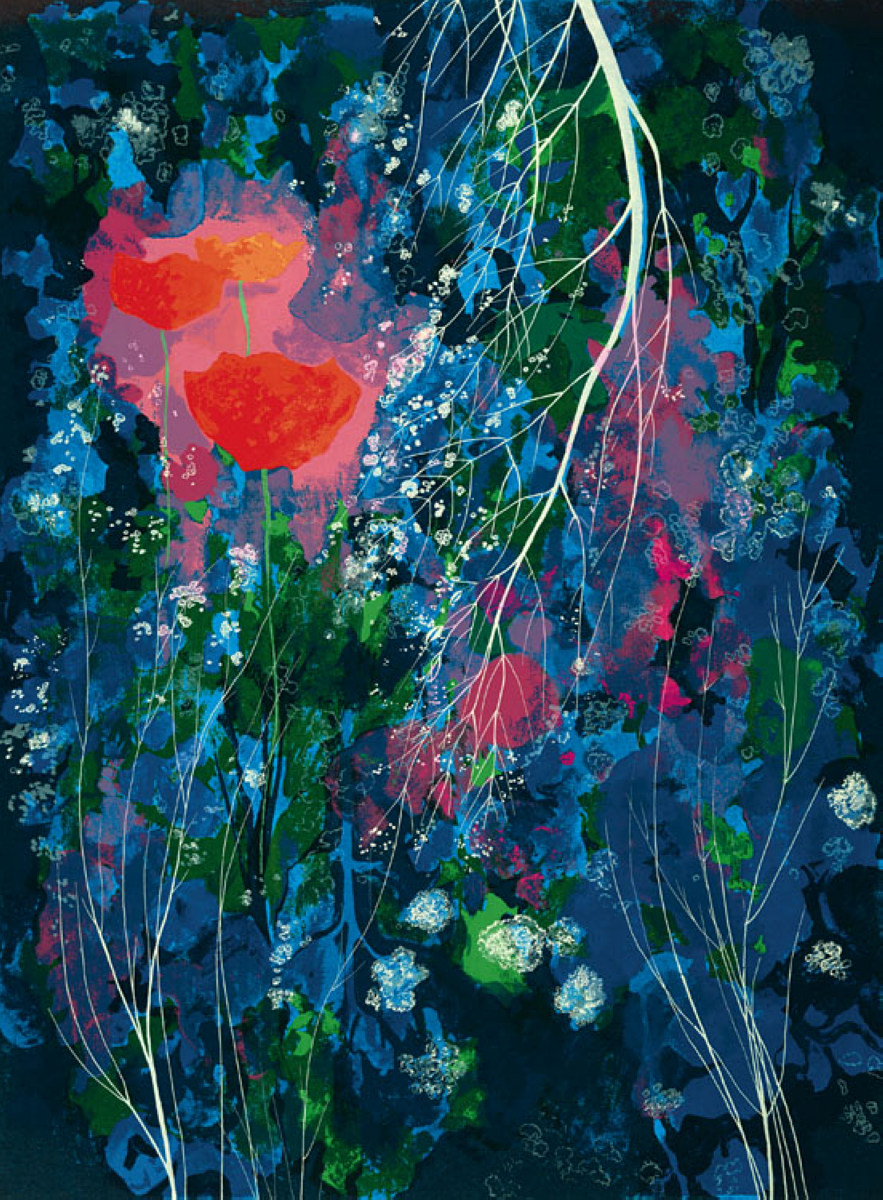This piece of art, titled "Poppies" from 1976, is an abstract oil on canvas filled with vibrant jewel tones set against a deep black background. The painting primarily depicts a flowerscape, with the background resembling a night sky. Dominating the composition are splashes and strokes of blue, turquoise, and sky blue, intermingled with shades of forest green and emerald green. Scattered throughout this dark and colorful expanse are bright reddish-orange poppy-shaped flowers, surrounded by pops of pink and flecks of white, which create an impression of poppies in bloom at night.

In the left third of the painting, there are three distinct red flowers with long green stems. Adjacent to these flowers, a white branch stretches down from the top, adorned with numerous smaller branches or wispy twigs. White vertical lines dispersed throughout the painting suggest the presence of trees. This abstract portrayal blends the elements seamlessly, with no definite top or bottom, creating an ethereal, almost dreamlike quality. The interplay of colors and shapes merges and blurs together beautifully, offering viewers a rich tapestry of abstract floral forms against a midnight backdrop.